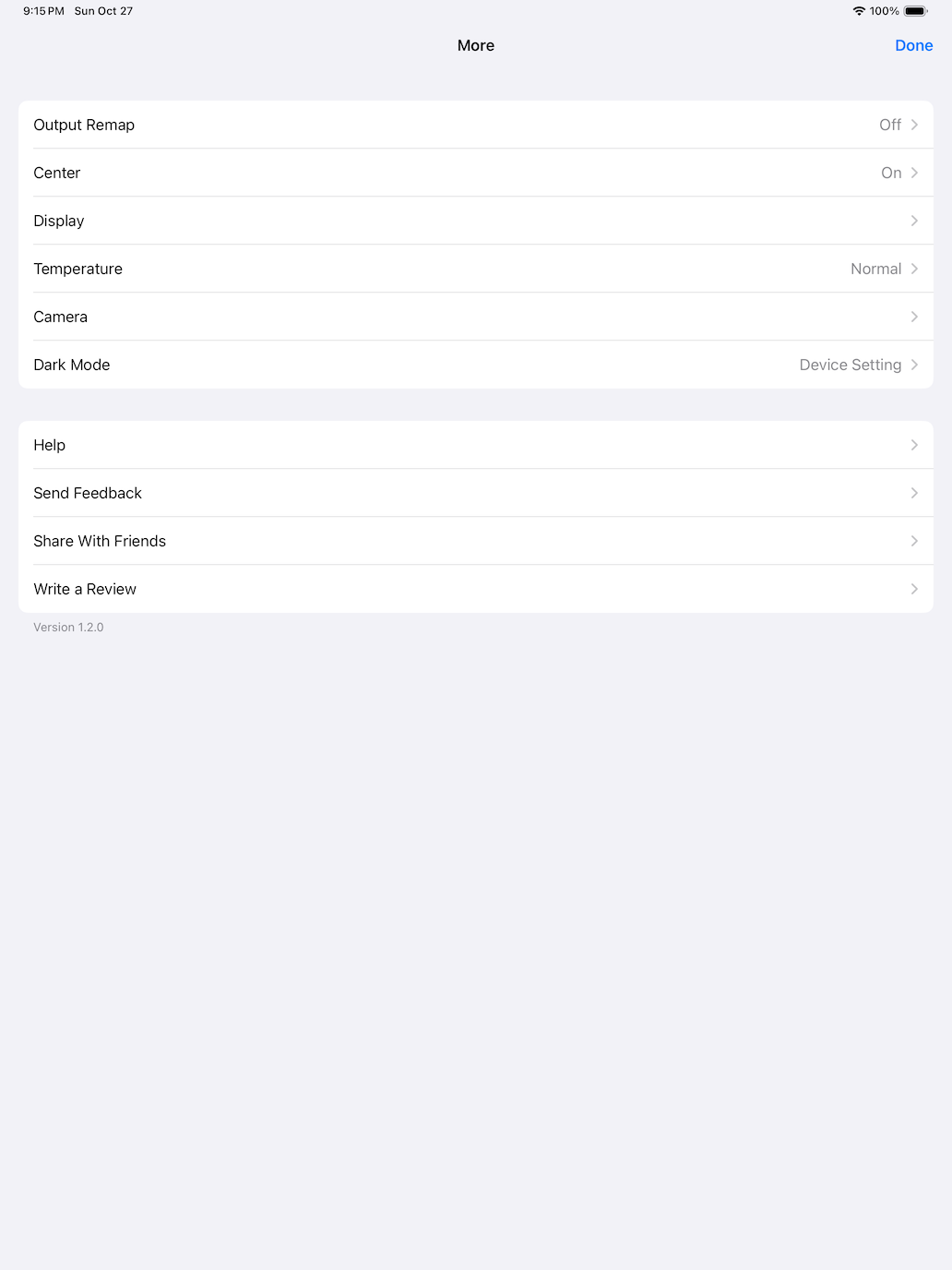A detailed and descriptive caption for the provided image could be:

---

In this image, we observe an interface from a phone application. The phone is fully charged with a battery level of 100% and has a strong Wi-Fi connection, as indicated by the full bars in the status bar. The current time displayed is 6:24 p.m. on Wednesday, February 2nd. 

The application features a sleek dark theme, with certain elements like the 'Refresh' and 'Done' buttons highlighted in a distinct blue color for easy visibility. The user interface includes several settings such as "XYZ", "Yaw", "Pitch", "Roll Output Remap", each with toggle options to switch them on or off. Currently, all these options are enabled except for "Output Remap" which is turned off. 

Below this set of options, there is another category with settings like "Center Display", "Temperature", and "Advanced Center". Within this category, "Center Display" is active, and "Temperature" is set to normal, while further details might be accessible by clicking the settings.

At the bottom section, the interface provides links to 'Help and Feedback', with arrows indicating that more information can be accessed by navigating further. The overall design maintains a grayish tone for text and elements on a predominantly black background, ensuring a visually balanced contrast.

---